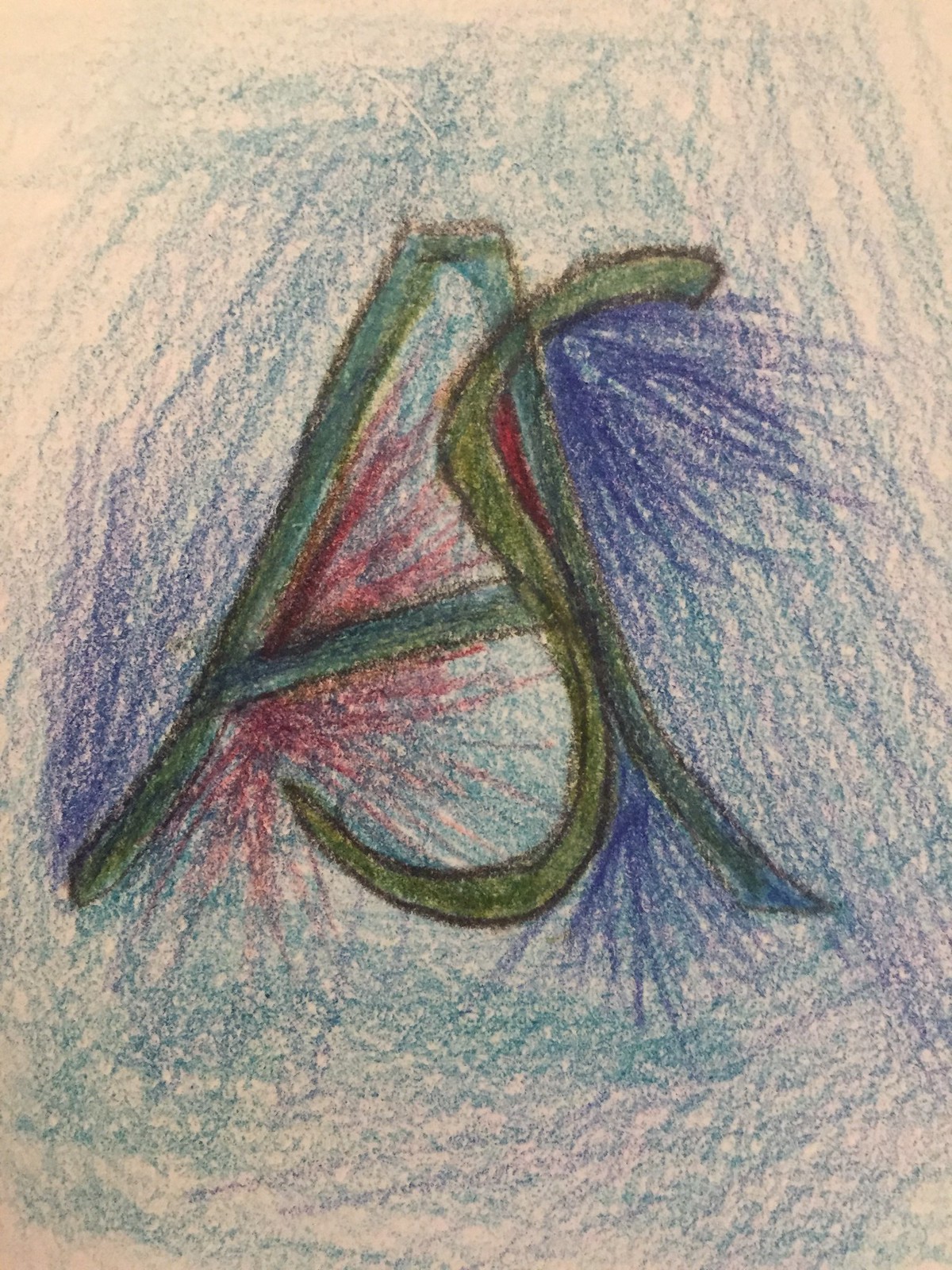The image features a whimsical children's drawing on beige paper, seemingly created with crayons. Central to the artwork are the letters "A" and "S", designed in a colorful, playful manner. The letter "A" is reminiscent of the California Angels logo, with its tapered shape that curves outward at the base and a crossbar that slopes at an angle of about 15 degrees from the lower left to the upper right. This "A" is primarily teal blue and positioned in the background. 

Overlaying the "A" is a vibrant green "S" with a central midsection that intersects where the crossbar and right leg of the "A" meet. Both letters are outlined in black, suggesting either preliminary guiding lines or intentional detailing. Surrounding the letters are a mix of blue and teal designs, with darker blue accentuating the inner top of the "A" and the space between the "A" and "S". Hints of red and white also sporadically embellish the background, enhancing the layered, dynamic composition.